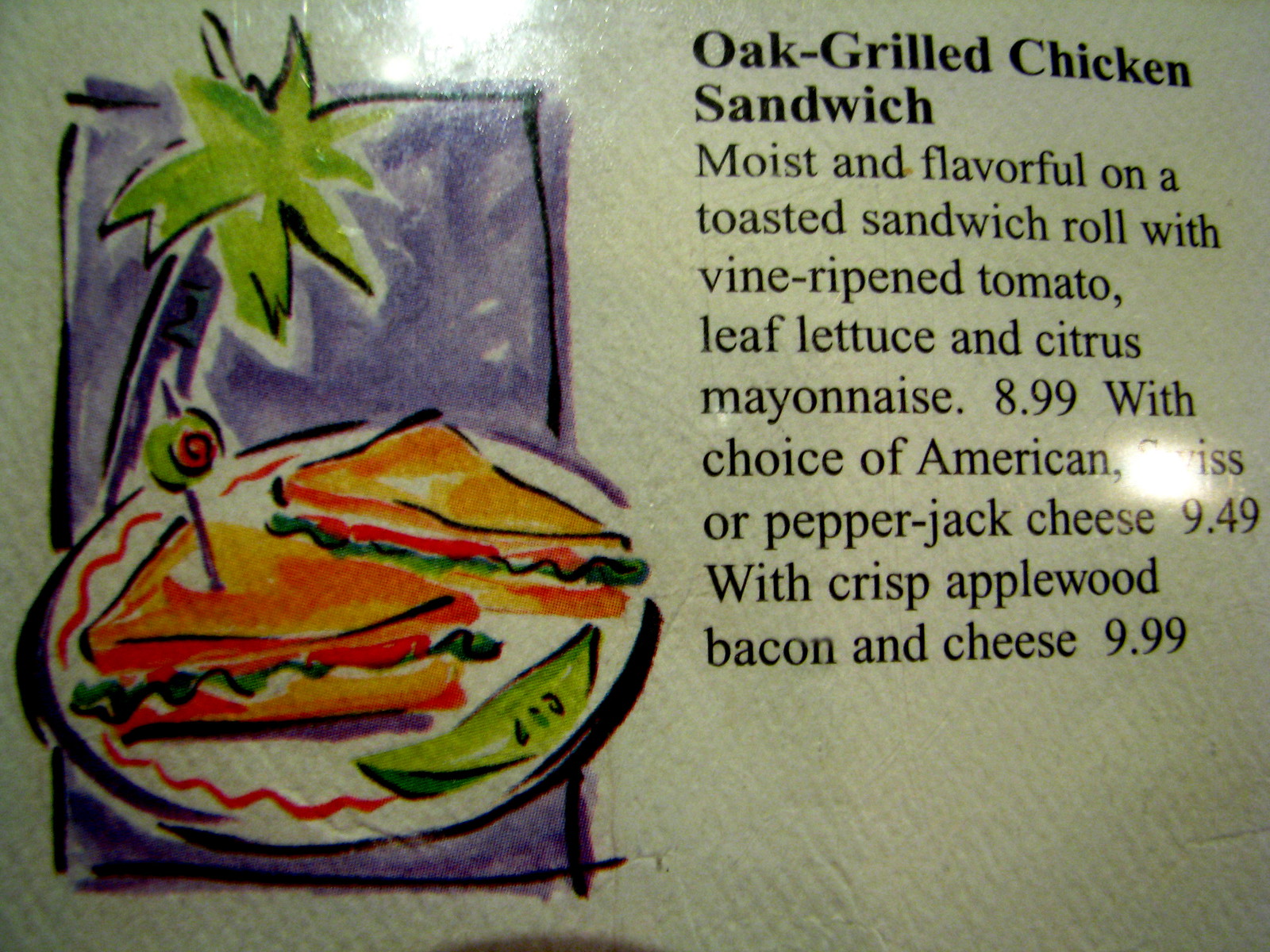This is a color photograph of a menu item, specifically highlighting a rectangular section that is slightly wider than it is tall. The image captures a single object from the menu with detailed clarity. At the top left, there is a subtle glitter effect, possibly from the camera flash or overhead lighting.

The left half of the photograph features a watercolor-like illustration with a predominantly blue rectangle framing the image. In the lower section, there is a plate holding a sandwich and a pickle. The sandwich is shown cut in half, with the lower piece skewered by a toothpick topped with an olive. Emerging from the left side of the plate is a whimsical depiction of a palm tree. The entire scene is set against a greenish background.

On the right-hand side of the photograph is the descriptive text for the menu item. In bold black letters spanning two lines at the top, it reads, "Oat Grilled Chicken Sandwich." Below this, in smaller but still dark and readable font, the description states: "Moist and Flavorful on a Toasted Sandwich Roll with Fine, Ripened Tomato, Leaf Lettuce, and Church's Mayonnaise." The price is listed as $8.99. 

Additional options are presented further down: "With Choice of American, Swiss or Pepper Jack Cheese for $9.49, with Crisp Applewood Bacon and Cheese for $9.99." The description text extends toward the bottom of the page but does not quite reach it. Notably, there is a bright glare of light in the middle right of the image, right over the word "Swiss," which slightly obscures part of the text.